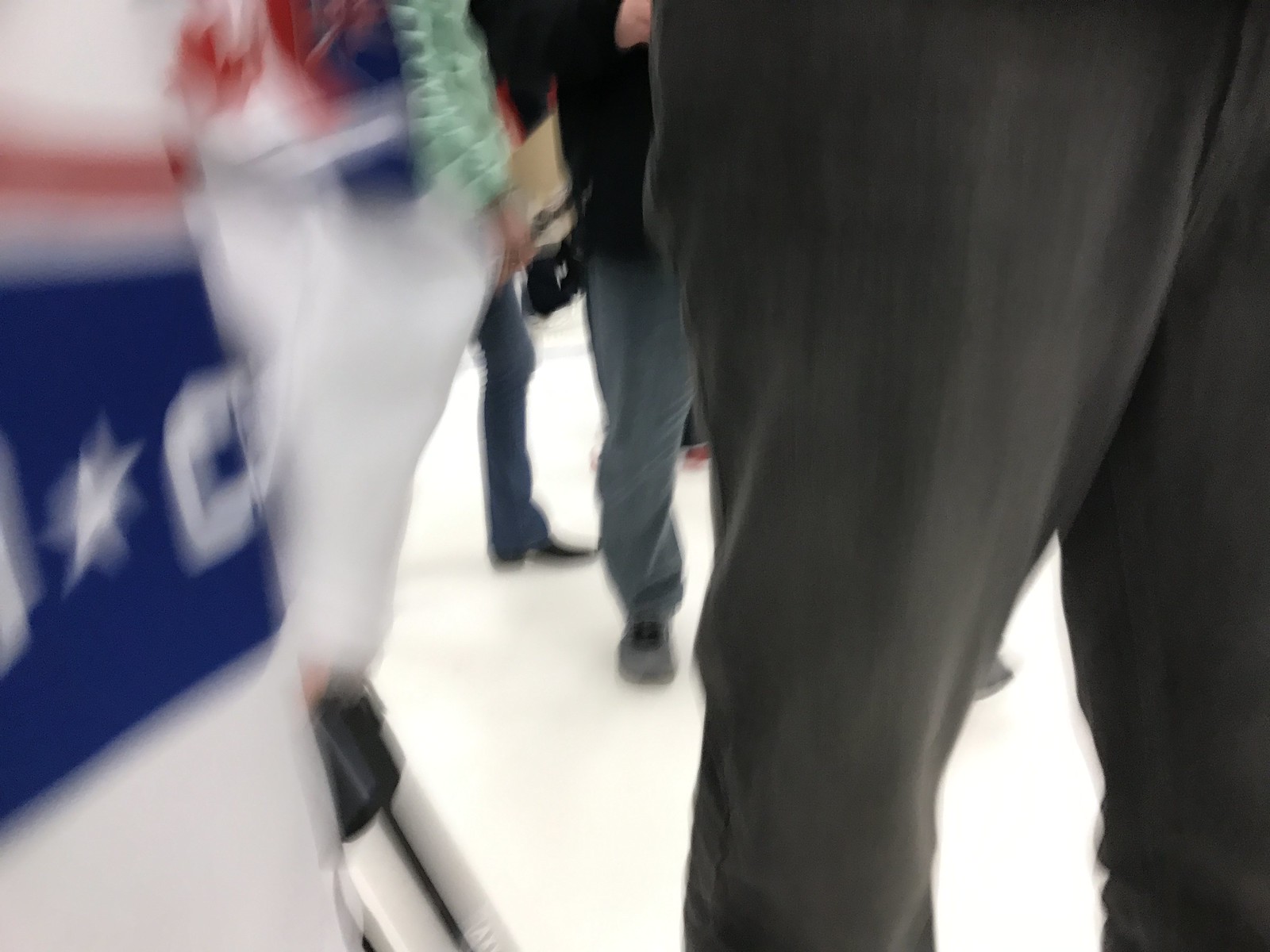This image is a blurry, out-of-focus photograph capturing the lower halves of a group of people standing on a smooth, white floor, which might resemble ice. Starting from the left, there's a close-up of a blurred blue, red, and white image that resembles either a campaign poster, a long hockey jersey, or potentially a bag. The image is primarily obstructed, showing white at the top, a red stripe, a large blue stripe with a star in the middle, and then more white. On the right side, we observe several individuals' legs: the nearest person wears grey dress trousers, while behind him there's someone in blue jeans and grey sneakers with a visible hand or wrist. Further back, a person's left leg is clad in tight blue jeans with brown boots, indicating a woman. Adding to the clutter, there seems to be a black purse with a visible strap in the background. All individuals appear to be standing in a line or walking away from the photographer.